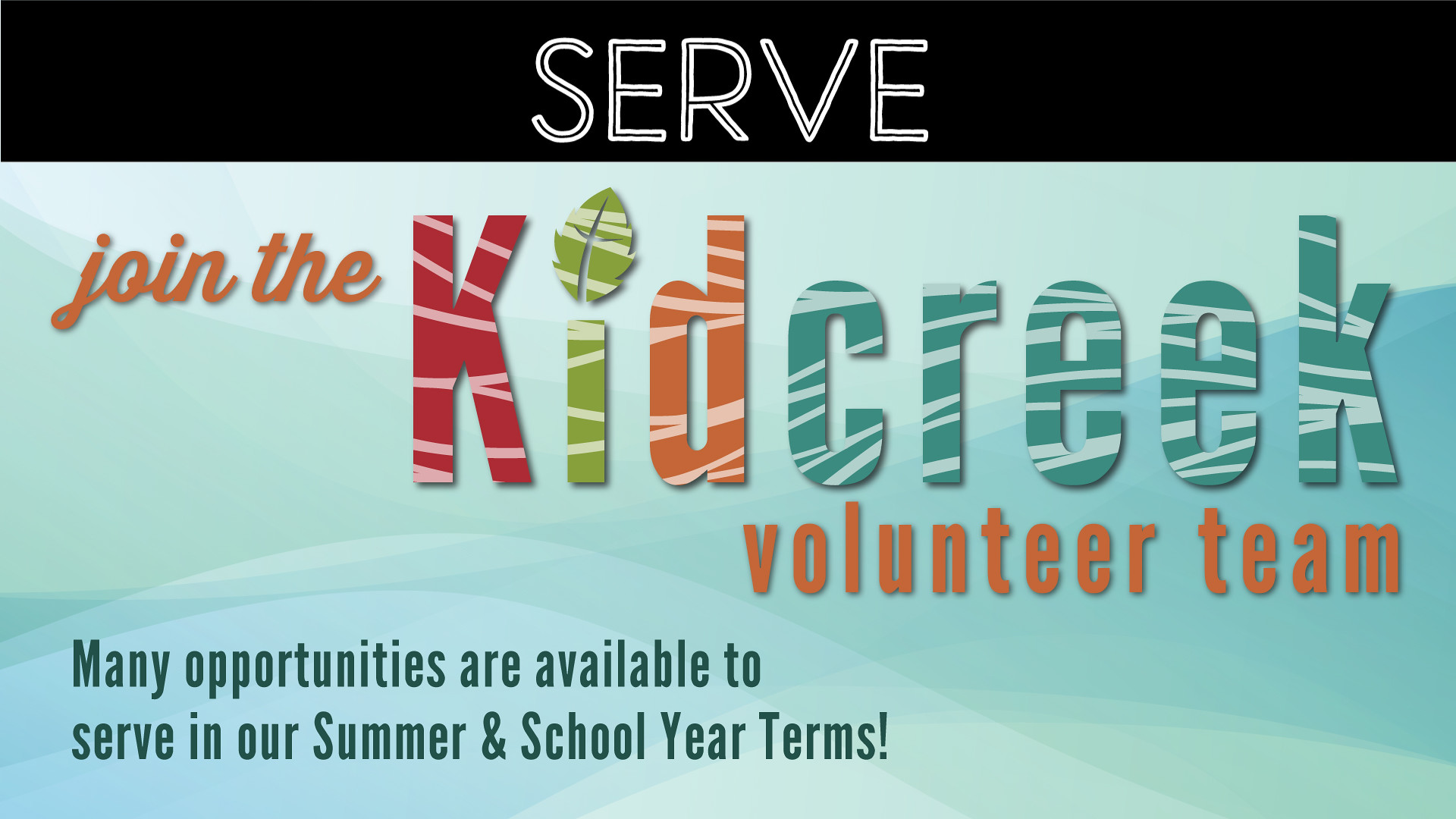This advertisement features a dynamic and colorful design. At the very top, a black rectangular section prominently displays the word "serve" in bold, white letters. The background of the bottom two-thirds showcases a blend of light blue, light green, and robin egg blue colors, creating a visually appealing palette. Centered in the image, vibrant text invites viewers to "join the Kid Creek volunteer team." The words "Kid Creek" are uniquely styled: the K is red, the I is green with a leaf as the dot, the D is orange, and "creek" is a lighter blue with white stripes resembling a zebra pattern. The phrases "join the" and "volunteer team" are written in orange, adding to the colorful scheme. In the bottom left corner, black text informs viewers that "many opportunities are available to serve in our summer and school year terms."